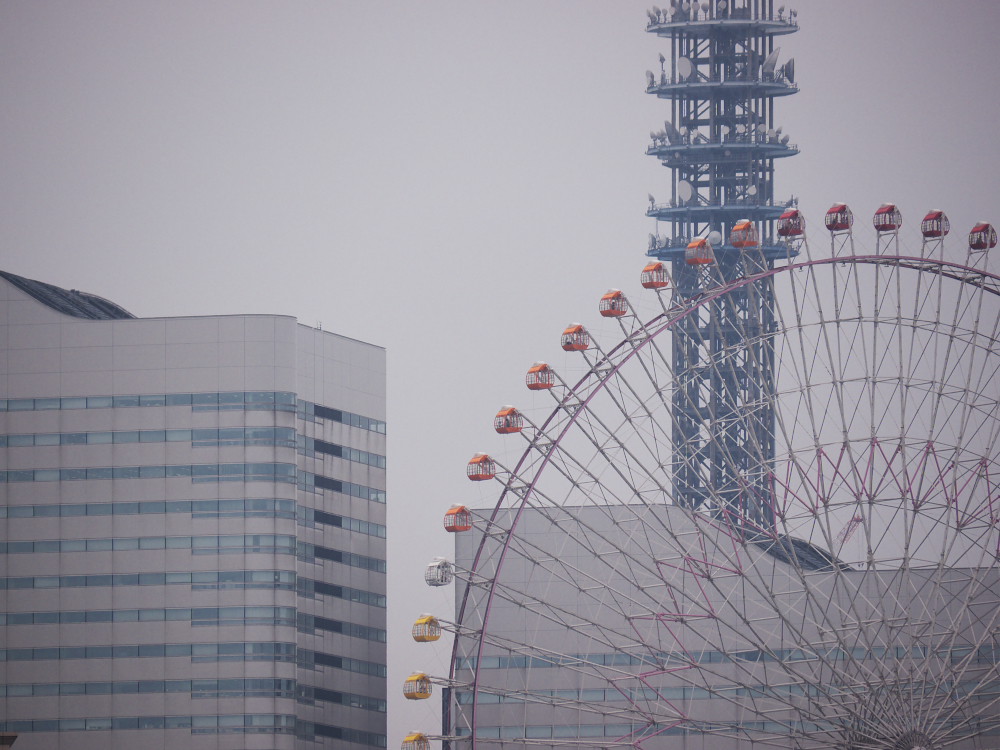The photograph, taken from an aerial perspective on a misty, foggy day, features a large, prominent Ferris wheel situated in the lower right section of the image. This Ferris wheel extends from the bottom center to the right center, displaying cars in shades of yellow, white, orange, and red, each adorned with some form of printing. The Ferris wheel appears stationary and devoid of passengers. Adjacent to the Ferris wheel, on both the left and right sides of the image, are multi-story buildings with numerous glass windows suggesting considerable height, possibly as tall as the Ferris wheel itself. Behind the Ferris wheel, a tall, skeletal tower is visible; it includes several small platforms and what appear to be satellite dishes or reception dishes, enhancing the industrial or communications-oriented nature of the structure. The overall tone of the image is muted and gray, contributing to a somewhat somber and atmospheric setting.